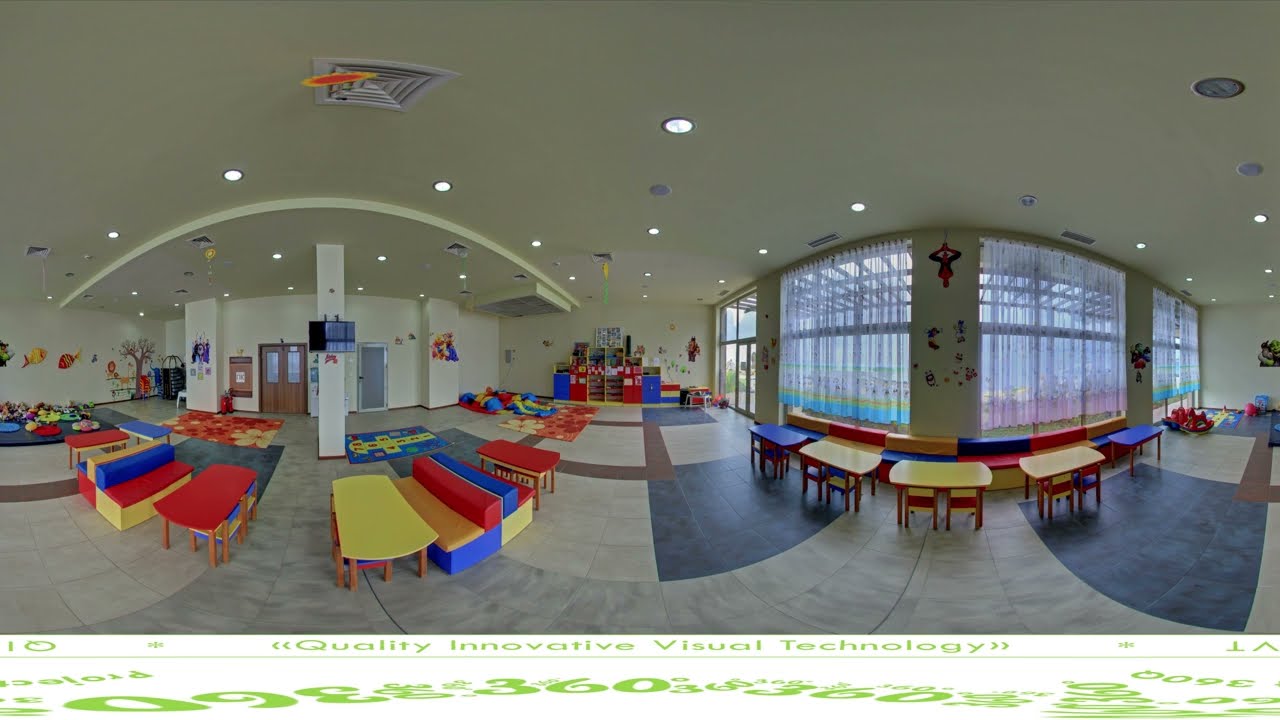The image depicts a vibrant and colorful children's play area, captured with a panoramic or bubble-like view. Dominating the foreground is a series of multi-colored tables and booths that form a U-shape, looping from the bottom towards the back of the room. These tables display an array of hues, with yellow tabletops and orange legs, complemented by blue roofs, encapsulating a playful and dynamic atmosphere. 

On the ground, the left side features mats in orange, red, and yellow, while a blue mat is positioned on the right, adding to the overall lively ambiance. The floor beneath these elements is presented in a white and blue checkered pattern, further enhancing the vibrant feel of the room. 

The perimeter of the play area is adorned with various decorations and toys scattered across the floor. The left-side wall hosts colorful fish designs, adding an element of aquatic fun, while centrally located shelving units offer storage against the white walls. 

To the right, additional tables continue the U-shape configuration, accompanied by a continuous bench that wraps around the corner of two walls, creating a cozy nook. This area is framed by large, clear windows adorned with sheer curtains, allowing ample natural light to flood the space. Adjacent to the windows, there are glass doors providing access to an outdoor area, as well as double doors on the left leading to another indoor section. 

The ceiling, painted white, is fitted with ceiling vents and lights, ensuring a well-lit environment. A support beam is also visible in the center of the room, contributing to the structural design of the space. This meticulous arrangement of colors, furnishings, and architectural elements collectively paints a detailed picture of a bright, engaging, and well-equipped children's play area.